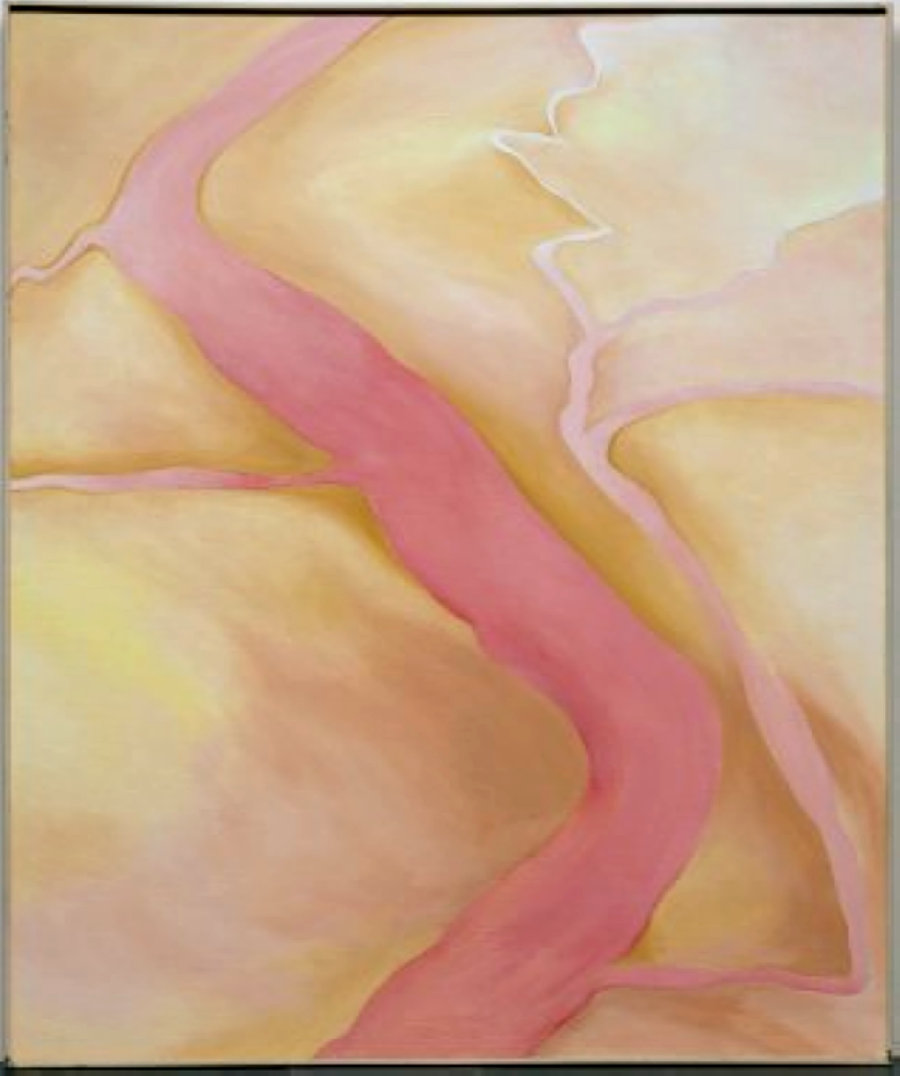This painting, in an abstract and impressionistic style, features a central red river meandering through a brown and yellow landscape. The river forms an S-shape, starting wide at the top and narrowing as it progresses towards the bottom of the painting. The river's hue transitions from a darker pink in the middle and bottom sections to a lighter pink near the top. To the right of the main river, a stream originating from a lighter pink, almost white, body of water flows towards the bottom right corner, eventually feeding into the main river. The background consists of varied swabs of yellows, browns, pale pinks, and whites, giving the impression of a textured and layered terrain. Throughout the river's journey, it is interspersed with several tributaries: one in the top left, another crossing the river at its midpoint, and yet another towards the bottom right corner. The scene devoid of text, combines elements of watercolor and possibly oil painting to create a fluid and dynamic composition reminiscent of a capillary-like network.